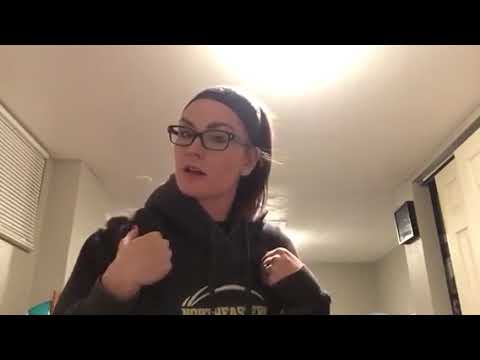The image is of a white woman standing in a beige-colored room, slightly left of center, with walls and ceiling of the same light beige shade. The camera angle is slightly tilted upwards, capturing her with her left side facing the camera. She is wearing a dark sweatshirt, either black or very dark brown, with a hood and two tassels hanging down her chest. The sweatshirt features a graphic on the chest, depicting a red curved arrow and yellow text underneath.

She has shoulder-length, straight brown hair, pulled back by a black headband. The woman is wearing rectangular, dark-rimmed glasses. Her mouth is slightly open, and her hands are clasped tightly in front of each shoulder, with her elbows bent. Above her, there is a light fixture on the ceiling, and another light source is visible in the distance behind her. The room's features include an air vent to the left, a small plaque on one of the walls, and a sliding door closet to the far right. Thin black stripes frame the photo horizontally on the top and bottom.